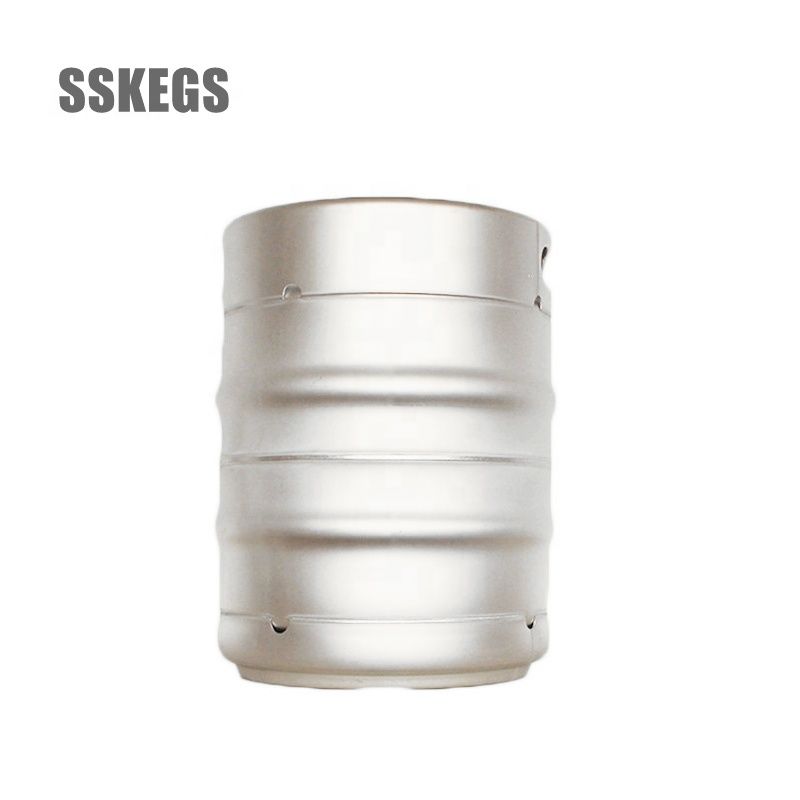The image features a prominently displayed, cylindrical, metallic object that closely resembles a keg, set against a stark white background. The keg's metallic silver color dominates the scene, enhancing its industrial aesthetic. Horizontally oriented grooves encircle the keg, with distinct lines positioned at the bottom, middle, and top, contributing to its structured appearance. The top part of the keg appears to act as a removable lid, while the bottom is flat, suggesting stability for ground placement. The overall height of the object is approximately three to four feet, implying a substantial, heavy build. In the upper left corner of the image, the bold, capitalized letters "SSKEGS" are emblazoned in dark gray, providing the only textual element on the otherwise unadorned surface. The simplicity of the design and background directs full attention to the product, hinting at a possible promotional context.